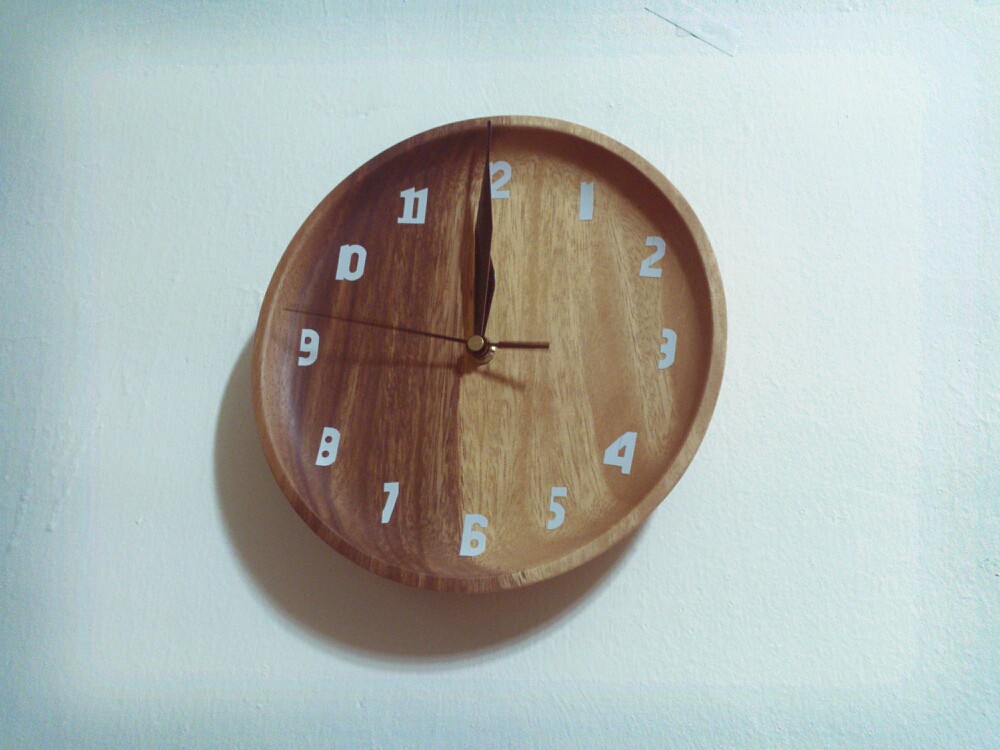This photograph captures a round, wooden clock mounted on a textured, white plaster wall. The wall's surface shows subtle variations, including some drips where paint has dried unevenly. The clock itself displays a striking contrast, with its left half featuring a darker brown wood stain and its right half, from the 12 to the 6 o'clock positions, showcasing a lighter wood stain. The clock's numbers are rendered in white, providing clear contrast against the wood, while its hands - hour, minute, and a slender second hand - are black. A soft shadow from the hands is visible on the clock face, and an additional shadow of the clock is cast on the wall below. The time indicated is precisely 12 o'clock.